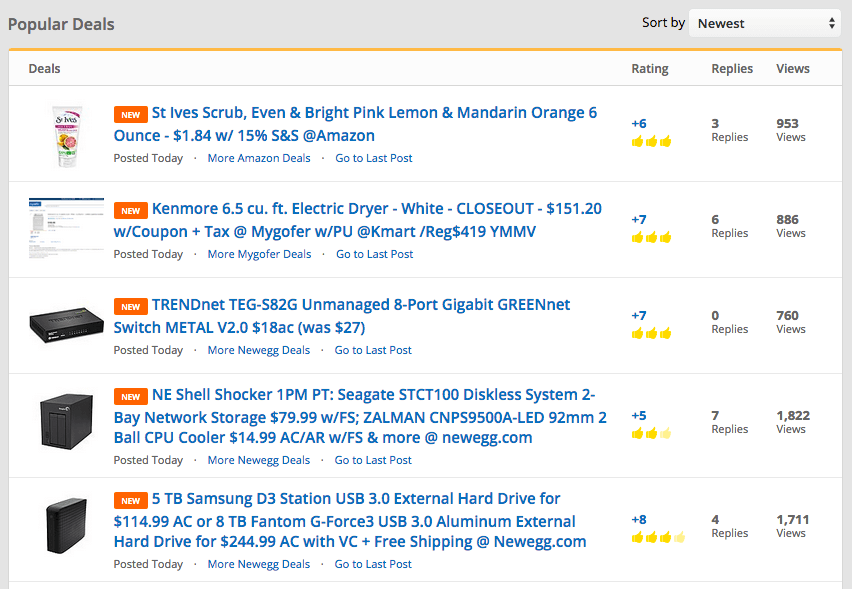This image depicts a website functioning as an aggregator for multiple deals, showcasing a variety of products under a "Deals" header. Featured items include:

1. **St. Ives Scrub**: Rated with three thumbs up, this product has garnered three replies and 953 views.
2. **Kenmore Electric Dryer**: Also rated three thumbs up, this deal has attracted six replies.
3. **Gigabit Green Net Switch**: With no replies but receiving three thumbs up, this network switch is also listed.
4. **Network Storage Bay**: The most viewed product among the list, it has attracted 1,822 views with an unspecified thumbs-up rating.
5. **External Hard Drive (8 Terabytes)**: With three clearly visible thumbs up and potentially a fourth one grayed out, this product has four replies.

Each item is succinctly detailed with user engagement metrics, highlighting their popularity and user interaction.